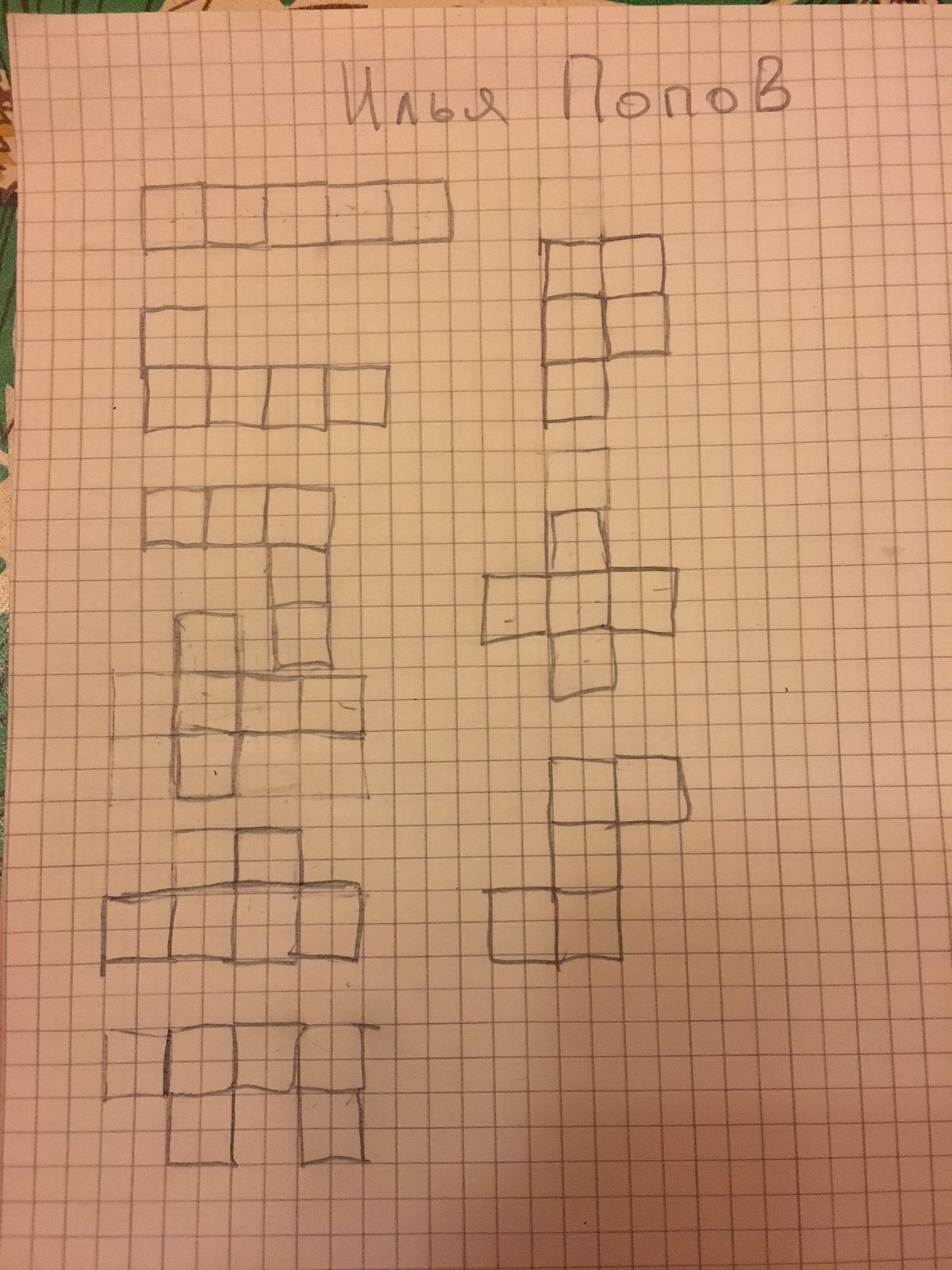The image showcases a piece of graph paper with Russian lettering visible at the top. Below the text, multiple grid designs are drawn in pencil, each showcasing various configurations of connected boxes. The first design features five boxes aligned horizontally. The second design displays four boxes aligned horizontally with an additional box positioned above the leftmost box. The third design consists of three boxes aligned horizontally, followed by two more boxes placed beneath the rightmost box of the initial three. The next design includes a horizontal row of three boxes, with an additional box situated above and below the leftmost box in the row. Below this, a horizontal arrangement of four boxes is depicted, with an extra box positioned above the third box from the left. The final design consists of a horizontal row of four boxes, where the second box from the right has an additional box below it, and the fourth box from the right also has an additional box beneath it.